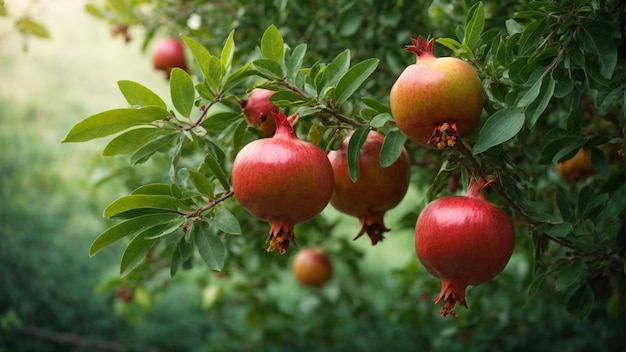This close-up photograph features a detailed view of several branches from a pomegranate tree, adorned with both ripe and partially ripe pomegranates. The prominently displayed pomegranates are large and onion-shaped, with a vivid reddish-gold hue, while others exhibit a mix of red and yellow, indicating varying stages of ripeness. There are five pomegranates in sharp focus in the foreground, vividly showcasing their attachment points to the branches. These branches are also lush with dark green leaves. The background is softly blurred, revealing additional pomegranate trees or bushes with smaller, less distinct fruits and lighter-colored leaves. A source of white light, possibly the sun, filters through the foliage, adding a subtle brightness to the scene. The abundance of fruit and verdant leaves paints a vibrant picture of a thriving pomegranate grove.